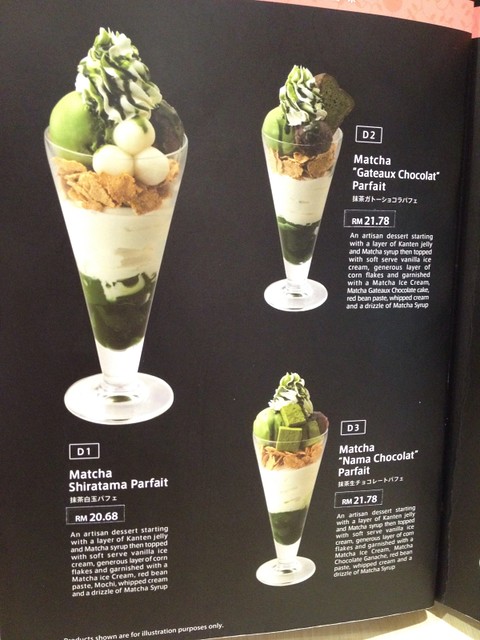This advertisement showcases three exquisite matcha parfaits against a solid black background, each meticulously labeled and accompanied by detailed descriptions and pricing information. Featured prominently are rich, vibrant photos of the parfaits, revealing their intricate layers and ingredients.

The first parfait, designated D1, is the Matcha Shiratama Parfait. This artisan dessert begins with a layer of kanten jelly and matcha syrup, followed by soft-serve vanilla ice cream. It includes a generous layer of crunchy corn flakes and is artfully garnished with matcha ice cream, red bean paste, matcha whipped cream, and an additional drizzle of matcha syrup.

The second parfait, labeled D2, is the Matcha Gateau Chocolat Parfait. Similarly described as an artisan creation, it features layers and components that highlight the combination of rich chocolate and earthy matcha flavors.

The final parfait, D3, is the Matcha Nama Chocolate Parfait. Like its counterparts, it boasts an intricate assembly that harmonizes creamy matcha with decadent nama chocolate.

Each parfait is presented in a clear, tall glass, showcasing its layered composition. The detailed presentation allows viewers to appreciate the exquisite craftsmanship and enticing ingredients of these delectable matcha parfaits.